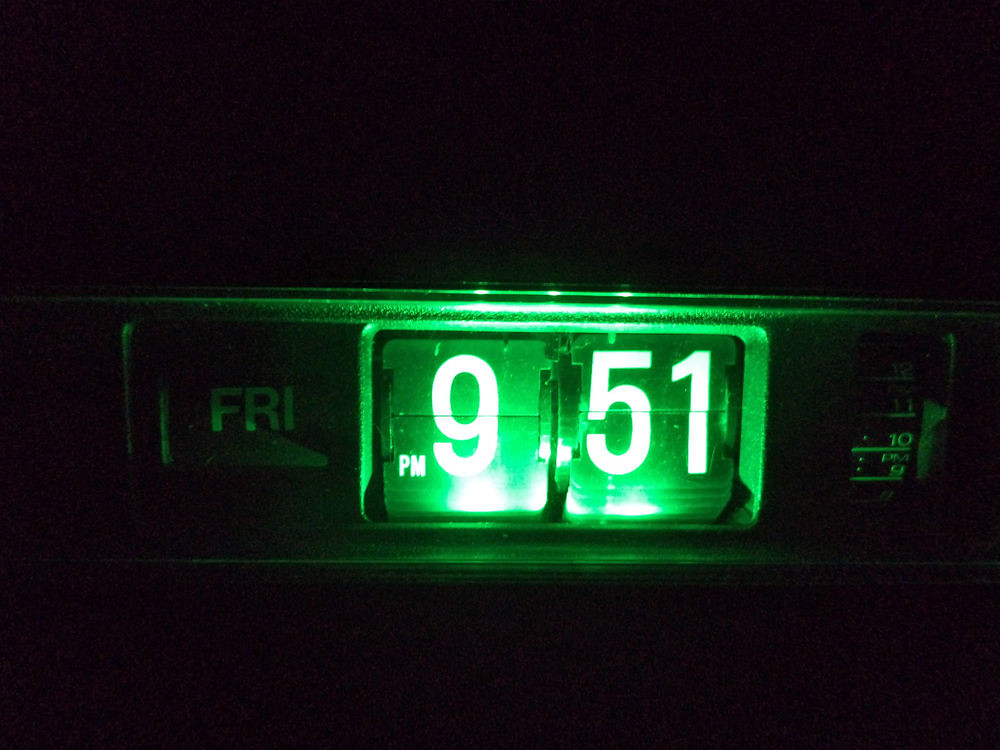In the photograph, an alarm clock is prominently displayed against a pitch-black background, creating a striking contrast. The clock itself is a horizontal rectangular shape and appears mostly black, although the illumination might give it a greenish tint. On the left side of the display, a small square indicates the day of the week with "FRI" for Friday. The central illuminated section clearly shows the time as 9:51 PM, with a large white "9" followed by "PM" and "51." To the right of the main display, there's a dial with visible numbers indicating the hours, starting from "12" at the top and descending through "11," "10," down to "9," with a faintly readable "8" beneath. The dial also seems to include an additional "PM" notation. The brightest and most prominent element of the image is undeniably the time display, reading 9:51 PM.